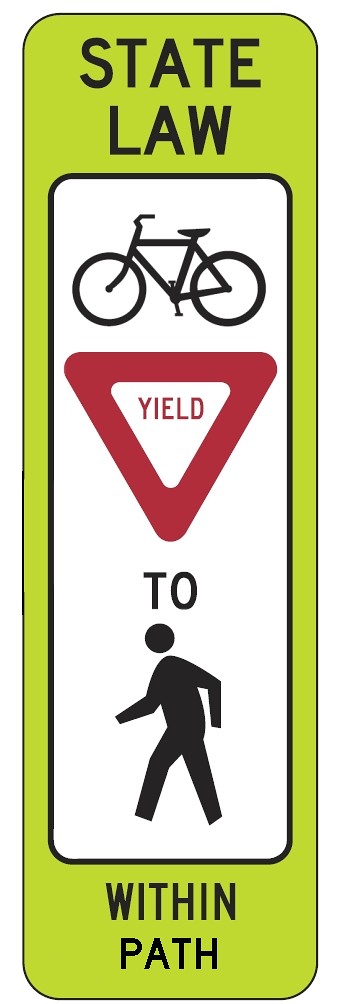The image depicts a tall, slender traffic sign with rounded corners and a green background. At the top of this green rectangle, there is bold black text stating "STATE LAW." Below, within the green rectangle, lies a smaller, black-bordered rectangle with a white background. Central to this white section are a series of symbols and text: a black silhouette of a bicycle, a red yield triangle bearing the word "YIELD" in its center, the word "to" in black, and the black silhouette of a pedestrian walking. At the bottom of the green rectangle, more black text reads "WITHIN PATH." The overall message communicated by the sign is that, according to state law, bicycles must yield to pedestrians within the designated path.